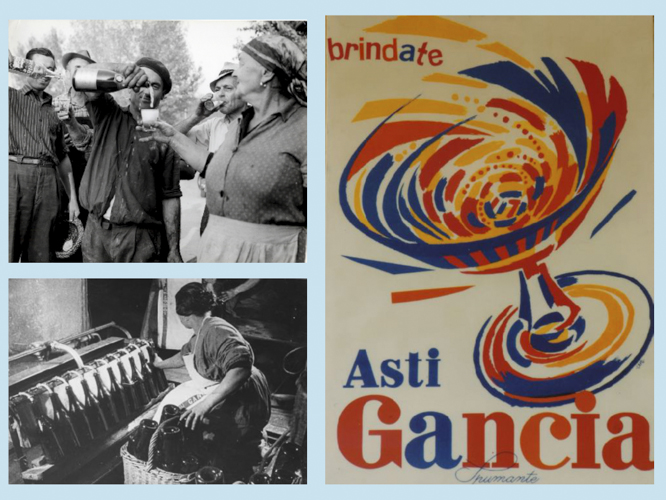The image is divided into three sections. On the right side, there's a colorful, impressionistic print ad with a blue border. At the top of the ad, the word "Brindate" is written, and at the bottom, "Asti Gancia" is displayed in cursive. The middle of the ad features a vibrant graphic of a martini-like glass with swirling colors of blue, yellow, and red. 

On the left side, there are two black-and-white photographs. The top photograph shows several people standing among trees. One man is pouring a liquid from a bottle into a glass held by an older woman. Another man, also pouring from a bottle, fills another glass, while a third man wearing a hat drinks from his glass. 

The bottom photograph shows a woman with brown hair, wearing an apron, sitting in front of a piece of machinery—possibly associated with the production process. She appears to be organizing bottles, which are grouped in a basket next to her.